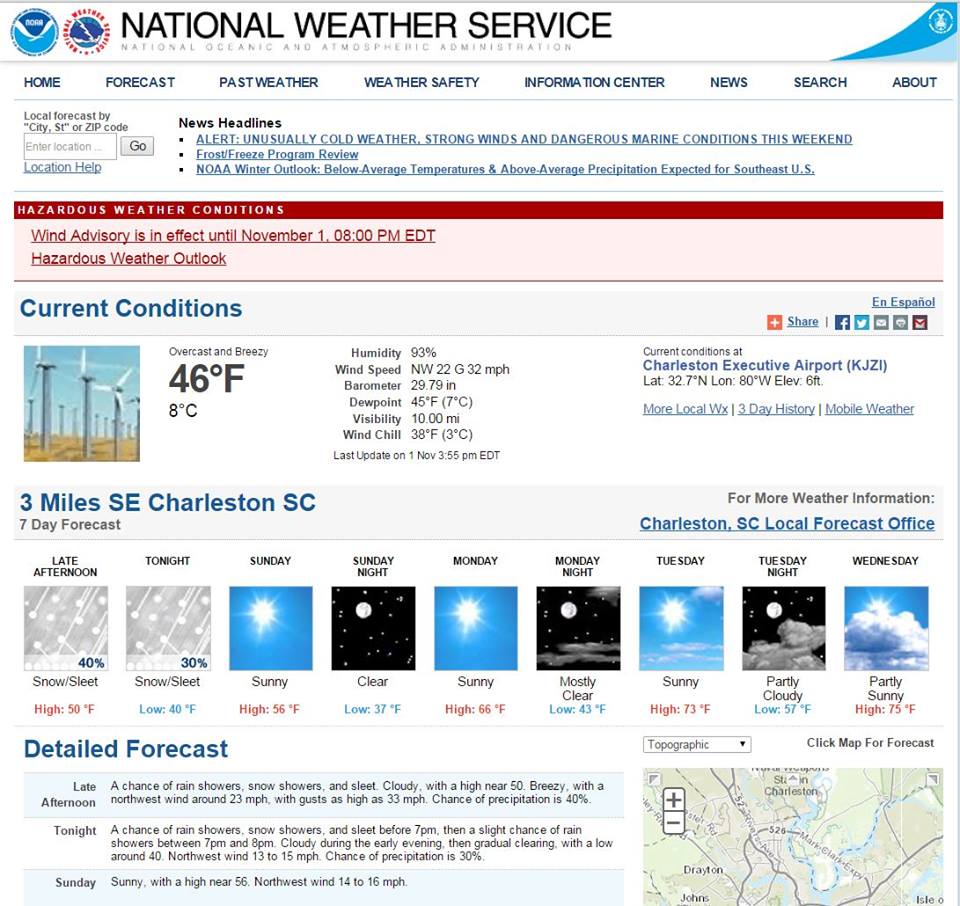**Screenshot of the National Weather Service Website**

The image shows a screenshot of the National Weather Service (NWS) website with a white background. In the upper left corner, there is a circular logo featuring a seagull and blue waves, representing the National Oceanic and Atmospheric Administration (NOAA). Below the logo, large black text reads "National Weather Service," and beneath it, in gray, it states "National Oceanic and Atmospheric Administration."

On the right side, there is a blue sidebar with various sections in both dark and light blue shades. The sections are labeled with black text and include options such as "Home," "Forecasts," "Past Weather," "Weather Safety," "Information Center," "News," "Search," and "About." Further down, black text prompts users to "Locate forecast by City/ST or Zip Code," next to a white search box with a gray "Go" button.

In the main content area, black text reads "News Headlines" with several blue, underlined links beneath it. A red notification indicates an advisory with the text "One advisory in effect until Nov 1, 8:00 PM EDT." A blue section labeled "Current Conditions" provides updated weather information: the temperature is 46°F, with a humidity of 93%. This particular forecast pertains to the Charleston Executive Airport, highlighted in blue.

Below the current conditions, there are blue icons representing different weather forecasts such as sleet, snow, rain, and sun. A detailed forecast is presented in black text, elaborated more extensively in a section titled "Detailed Forecast" in blue. Towards the bottom right corner, a Google Map shows the location related to the weather information provided.